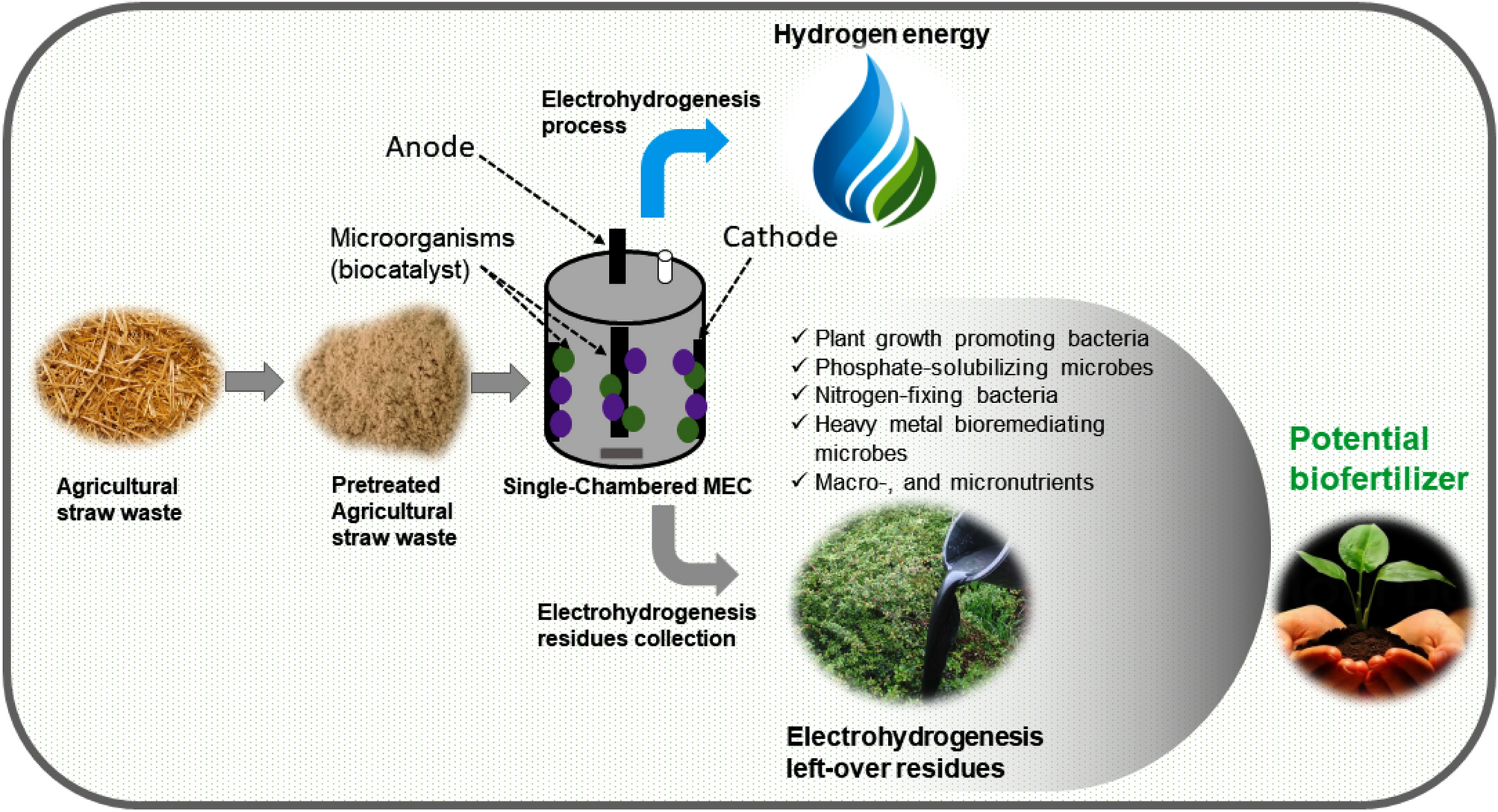This image depicts a detailed flowchart enclosed within a black-bordered rectangle with rounded corners on a white background. The process begins on the far left with agricultural straw waste, which then undergoes pre-treatment, resulting in a finer, dull brown version of the straw. This pretreated straw waste is then introduced into a single-chambered microbial electrolysis cell (MEC) where microorganisms (depicted in purple and green) act as myocatalysts. A node and cathode are labeled within this section, indicating critical components of the electrohydrogenesis process. This process converts part of the material into hydroenergy, symbolized by a half-blue, half-green teardrop image, while the remaining electrohydrogenesis residues are collected. These residues, containing plant growth-promoting bacteria, phosphate-solubilizing microbes, nitrogen-fixing bacteria, heavy metal bioremediating microbes, and essential macro and micronutrients, are depicted with checkmarks. Finally, the residual material is highlighted at the bottom of the chart as potential biofertilizer, illustrated by an image of a hand holding a plant with soil, emphasizing its application in agriculture.